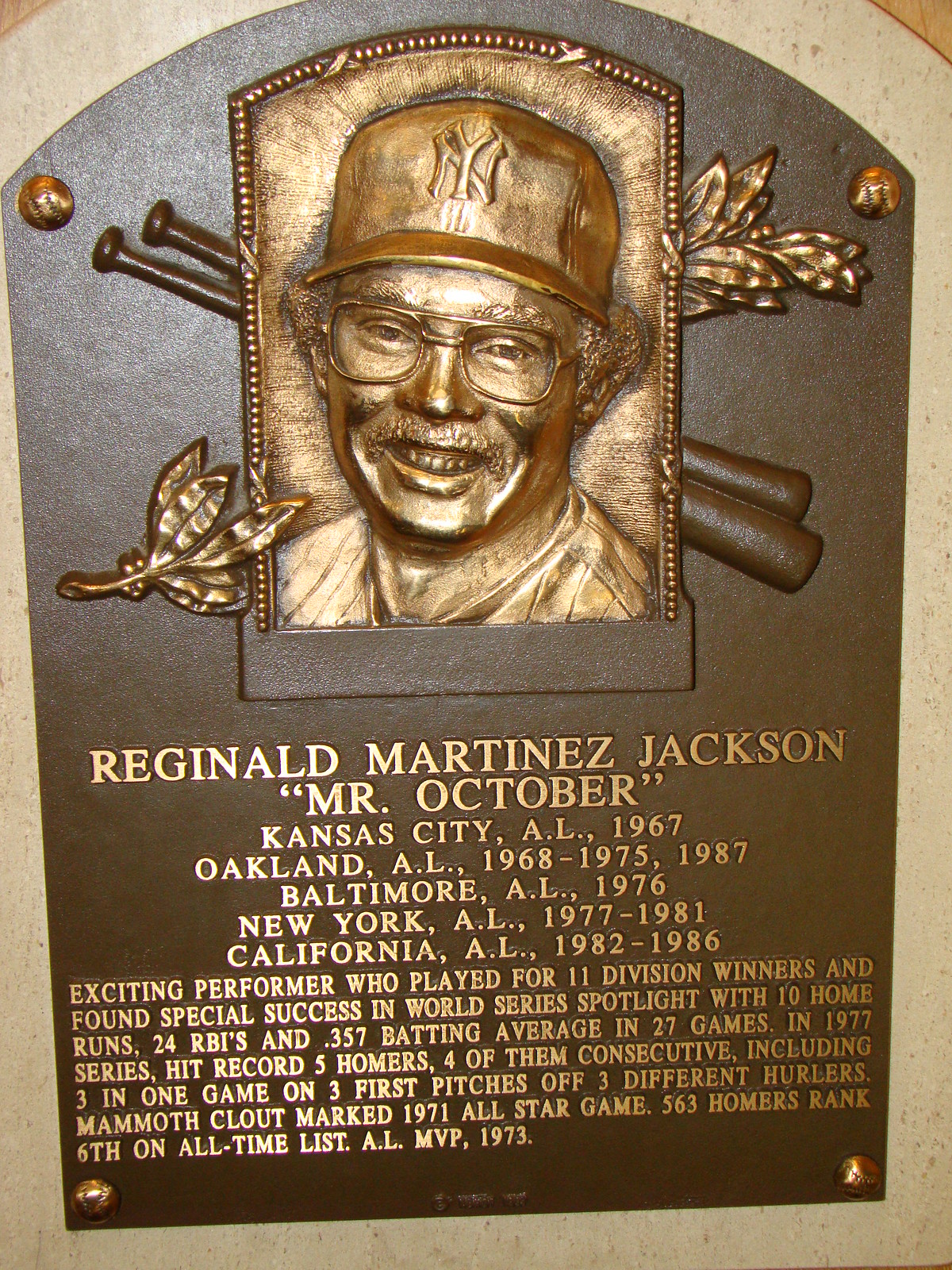This is a detailed photograph of a commemorative plaque honoring the illustrious baseball player, Reggie Jackson. The plaque is in the shape of a shield, with a curved top edge and straight bottom angles. Mounted to the wall with screws designed to look like baseballs, it features a raised, bronze-like sculpted relief of Jackson in the center. He is depicted wearing a Yankee cap, glasses, and has a warm smile on his face. Two baseball bats cross behind his image, complemented by leaf designs at the top right and bottom left.

Below the portrait, in gold relief, it reads: "Reginald Martinez Jackson, 'Mr. October'." The plaque meticulously lists his career details across various teams in the American League:
- Kansas City, AL, 1967
- Oakland, AL, 1968-1975, 1987
- Baltimore, AL, 1976
- New York, AL, 1977-1981
- California, AL, 1982-1986

A commemorative blurb highlights his remarkable achievements: "Exciting performer who played for 11 division winners and found special success in World Series spotlight with 10 home runs, 24 RBIs, and a .357 batting average in 27 games. In the 1977 series, he hit a record five homers, four of them consecutive, including three in one game on three first pitches off three different hurlers. Mammoth Clout marked the 1971 All-Star game. 563 homers ranked sixth on all-time list. AL MVP 1973."

The plaque's metallic and gold-tone finish lends a regal aesthetic, making it an ideal homage to Reggie Jackson’s stellar career, potentially marking his inclusion in Cooperstown.